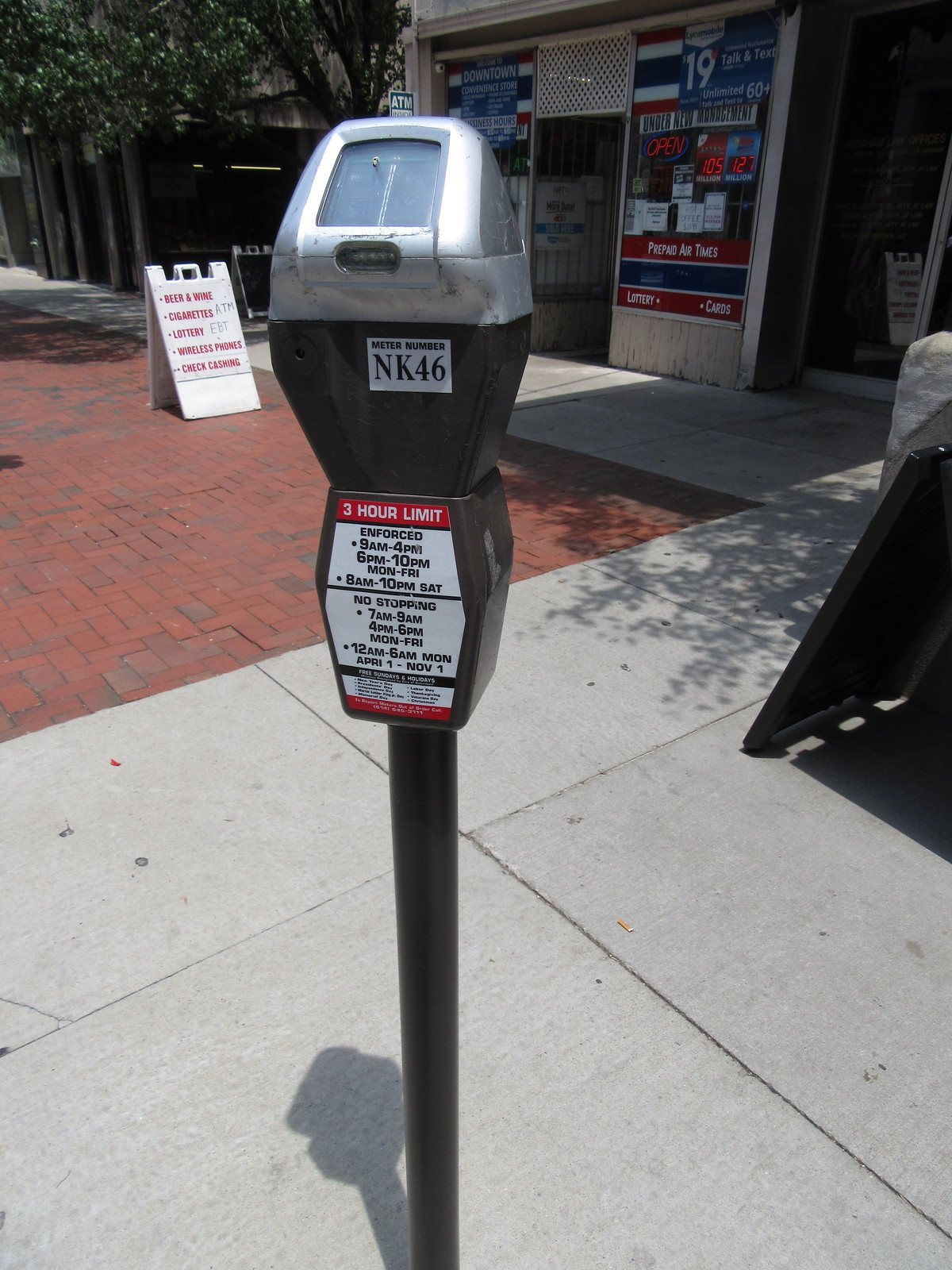This image captures a detailed scene centered around a parking meter, designated with the number NK46, situated on a gray cement sidewalk. The meter, featuring a black metal pole and a silver top with a blank gray screen, has prominent signage indicating a three-hour limit. The enforcement hours are specified as 9 AM to 4 PM and 6 PM to 10 PM from Monday to Friday, and 8 AM to 10 PM on Saturday. "No stopping" times are also noted from 7 AM to 9 AM, 4 PM to 6 PM Monday through Friday, and 12 AM to 6 AM on Monday from April 1st to November 1st. 

Adjacent to the sidewalk, there is a red brick pathway extending to the left. A prominent white A-frame board with red text is positioned on this brick area, advertising items like beer, wine, cigarettes, lottery, wireless phones, check cashing, and prepaid air times. 

In the background stands a storefront, identified as "Downtown Convenience Store," adorned with an array of vibrant signs and posters, both red and blue, promoting various items and services including lottery jackpots, talk and text plans, and an open sign indicating the store is under new management. The extensive use of text and neon signs creates a busy and colorful facade, enhancing the urban atmosphere depicted in the photo. 

Conclusively, the image portrays a typical urban setting where a well-detailed parking meter stands against a backdrop of a lively convenience store and its vibrant advertisements.